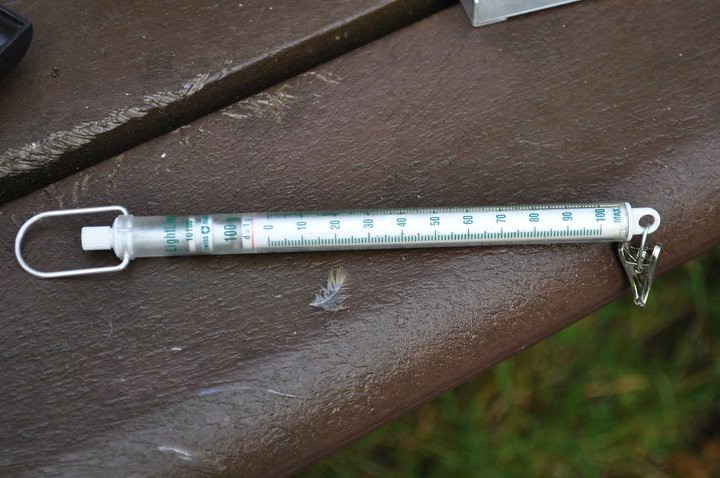The image depicts a small vial with green measuring marks ranging from 0 at the top to 100 at the bottom. Above the 100 mark, it also states "MAX" and "100". The vial features a symbol resembling a cross and shield. Inside the vial, there appears to be a white syringe with a hook at the top for gripping and a white loop with a metallic attachment at the opposite end. The vial is placed on a dark brown wooden bench photographed in close-up, making the background less clear. In the top left corner of the image, a black object is partially visible, while the top right corner shows a silver metallic object. Below the syringe is a feather, with blurred grass visible at the bottom of the frame.